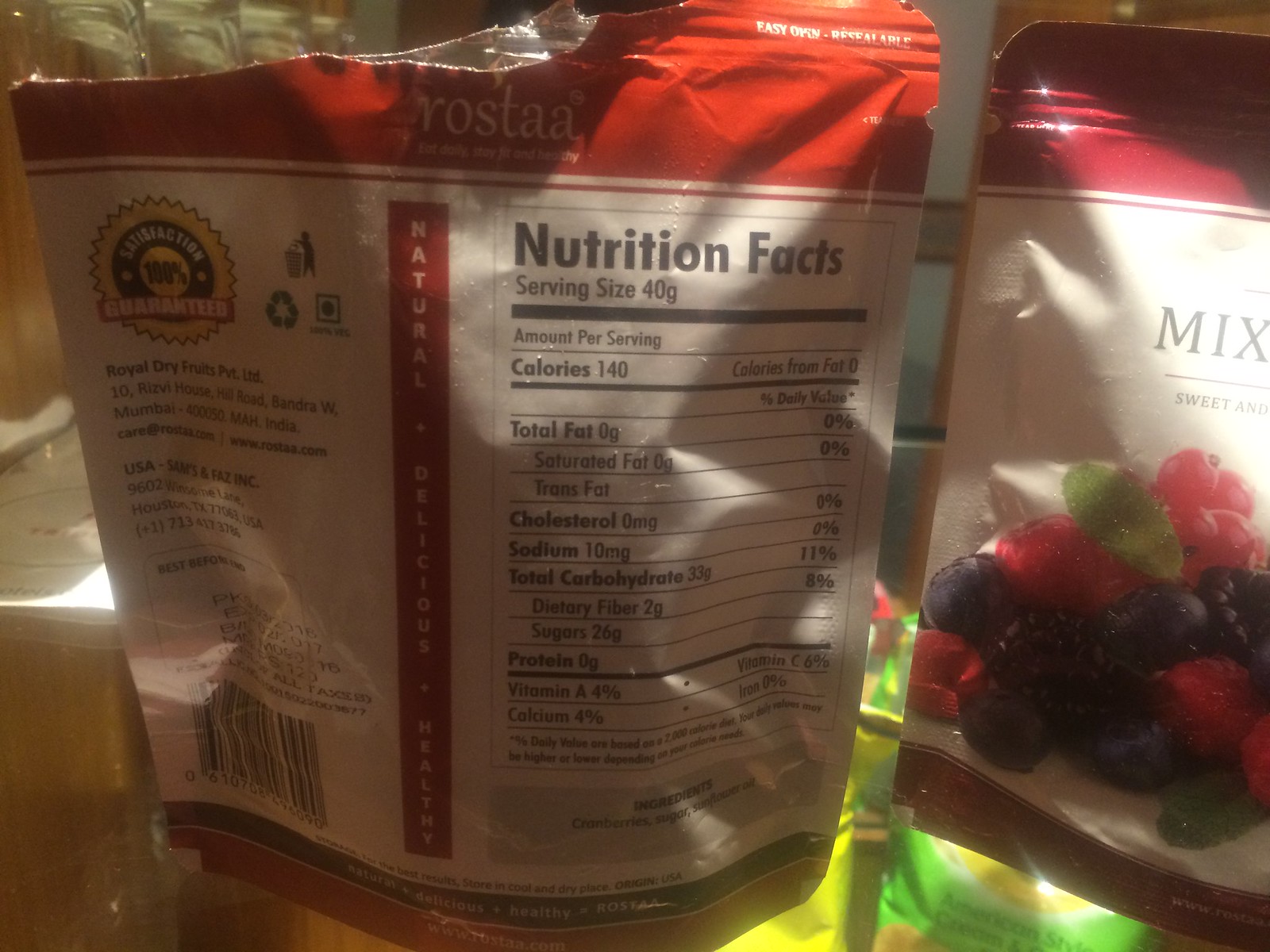In the center of the image, there are two bags prominently featured. The bag on the right has a distinctive red section at the top and displays a mix of black text indicating it contains sweeteners and other ingredients. This bag is partially obscured but remains mostly illuminated, unlike the other which is in shadow. In front of these bags, there's a vibrant pile of berries, including red cherries, green leaves, and blueberries. Appearing below this, hints of red fruit can be seen. The bottom left part of the image has text stating "American Style Theme" and additional details. On the left-hand side, the bag is already opened, with "Easy Open and Resealable" clearly marked at the top right. Below this, the brand name "Rosta" is visible, followed by the nutritional information: 40 grams per serving size, 140 calories per serving, 0 grams total fat, 0 grams cholesterol, 10 milligrams sodium, and 33 grams total carbohydrates. Text indicating "Natural" or "Delicious" (partially obscured) runs vertically along the side. A guarantee statement and a barcode are present on the top left.